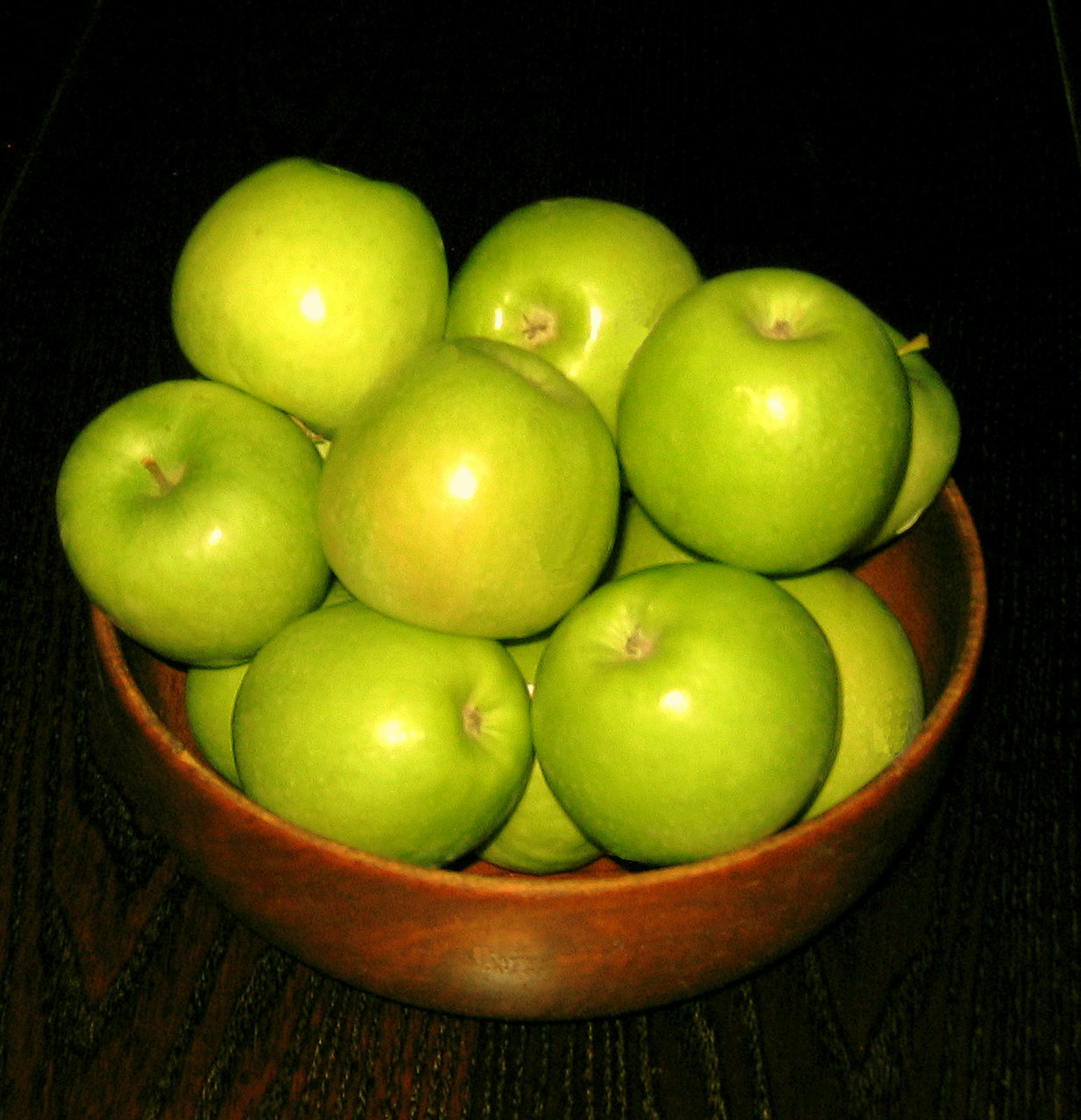The image showcases a wooden bowl, potentially made of cherry wood with a light brown, reddish hue, sitting on a table with a dark wood tone resembling mahogany. The tabletop's grain features distinct planks with varying groove patterns. Inside the bowl, there are approximately eleven to twelve green apples, tightly packed and facing various directions. Some apples have thin, narrow brown stems, with a few appearing slightly more rotted than others. The apples reflect light from a source behind the camera, illuminating their surfaces. The background is dark, making the detailed bowl and apples the focal points of the image.